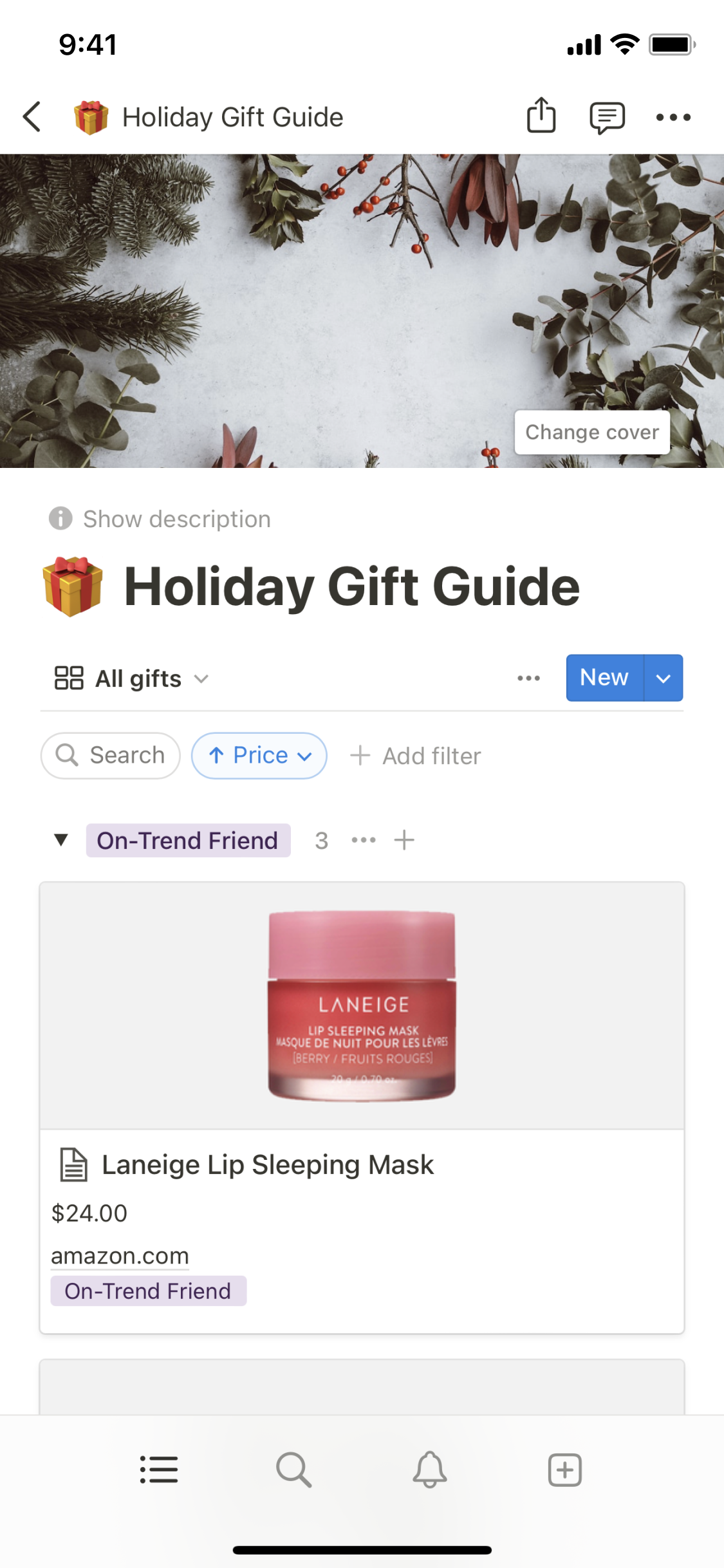Screenshot of an iPhone displaying a holiday shopping guide. The device shows a light background with a time stamp of 9:41 at the top, alongside four bars of cellular reception, four Wi-Fi bars, and a full battery icon. Below this, there is a header with a back arrow on the upper left corner, next to an image of a gift box with a red ribbon, labeled "Holiday Gift Guide."

Directly beneath this header, the main image showcases a snowy ground adorned with pine needles and red berries. A white button labeled "Change Cover" allows customization of this image. 

Further down, a larger version of the gift box image reiterates the title "Holiday Gift Guide." The page includes a selection tab currently highlighting "All Gifts," next to which is a blue button marked "New" with a drop-down menu icon.

The featured product displayed is the Laneige Lip Sleeping Mask, priced at $24, available on Amazon.com.